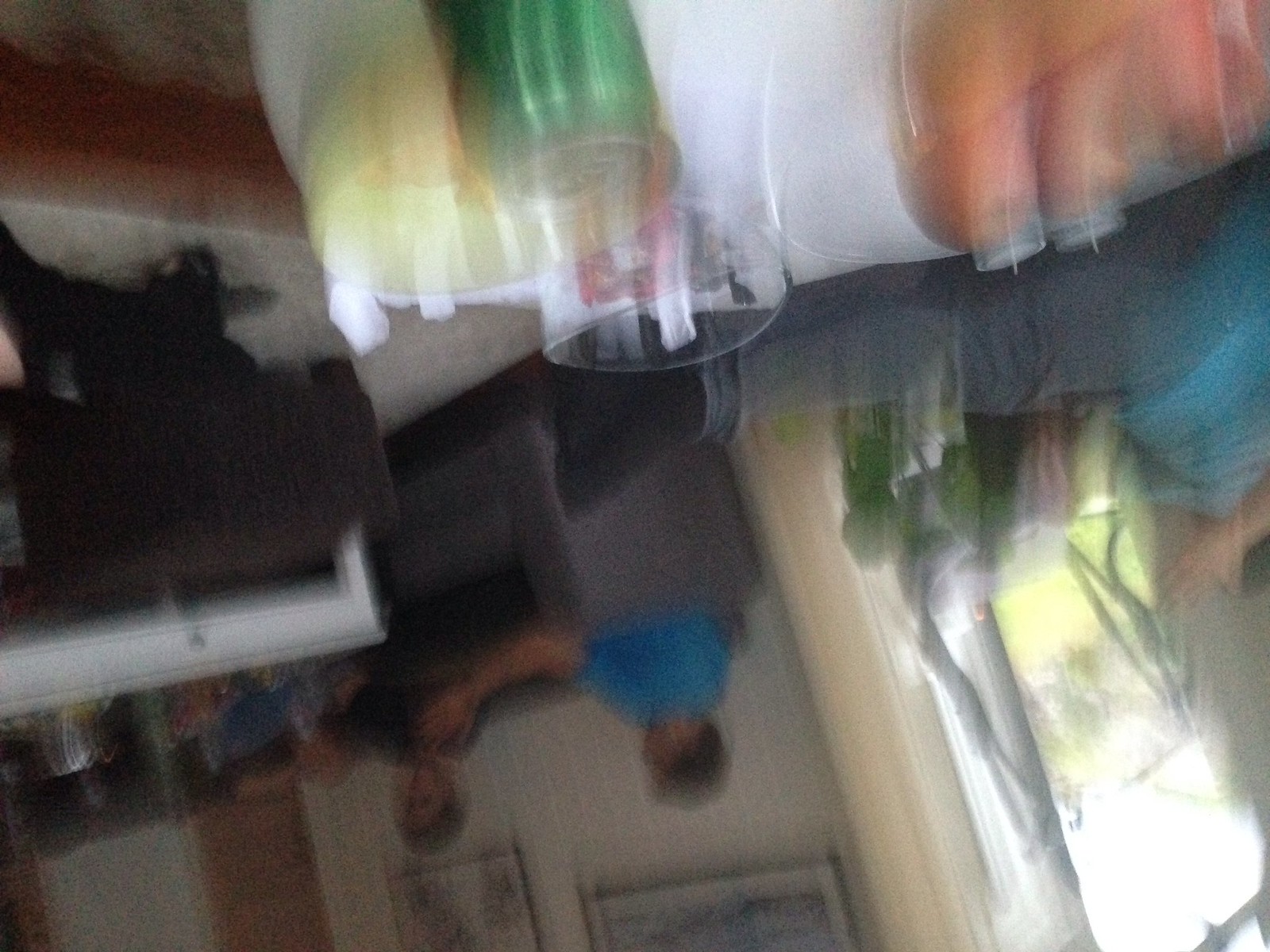Here is a cleaned-up and detailed caption:

"An accidentally captured and extremely blurry, upside-down photo of a home or apartment interior. Despite the distortion, one can discern a table in the foreground cluttered with glasses and drink cans. In the background, through another room, a grey couch is visible with two people seated on it—one in a blue shirt and the other in a black shirt. Behind them is a white wall adorned with framed wall art. The overall impression is chaotic due to the image's poor focus and orientation."